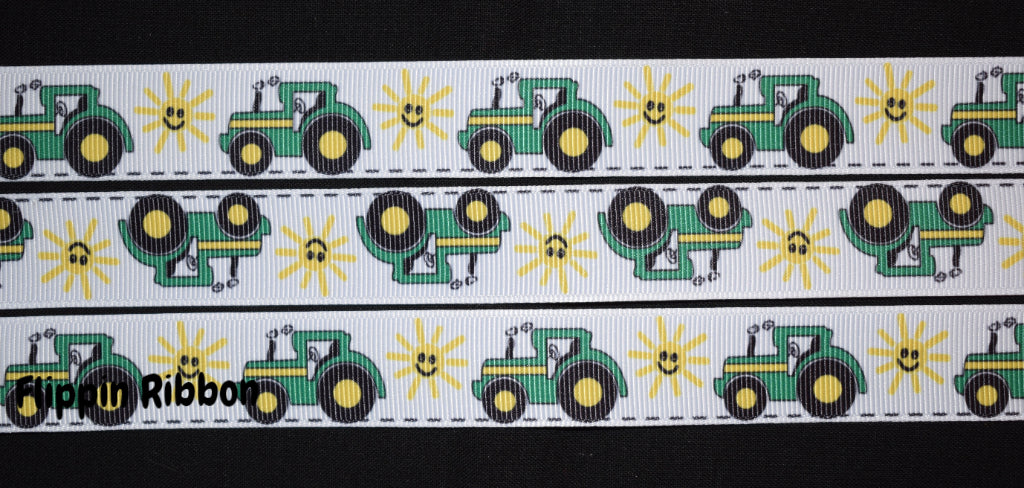This image showcases three sections of a whimsical ribbon laid out against a black background. The ribbon is organized with the top and bottom sections positioned right side up and the middle section flipped upside down. The ribbon itself is primarily white and features a playful pattern repeating green tractors and yellow suns with smiley faces. Each tractor has black wheels with yellow centers and a yellow stripe at the bottom, and is depicted emitting small puffs of smoke from the exhaust. The suns are simple yellow circles with radiating lines and a cheerful face. Running along the bottom edge of the ribbon is a black dashed line, giving the impression of a road. In the lower left corner of the image, the text "Flippin' Ribbon" appears in a subtle black font that nearly blends into the background.